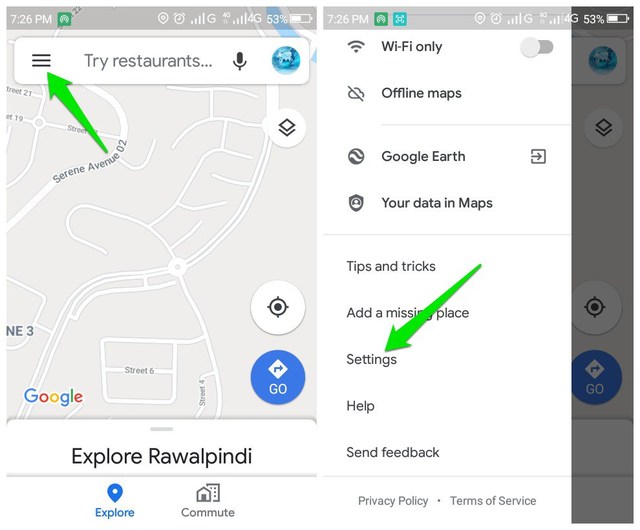This image showcases the mobile version of the Google Maps app. Overlaying the map are two green arrows that have been drawn onto the image. The first green arrow directs attention to the three lines (commonly known as the "hamburger menu") located next to the search bar at the top of the screen. The second arrow points to the settings icon on the left side of the screen. On the right side of the image, a neighborhood map is visible with the label "Explore Rawalpindi" beneath it. Additional menu options include "Wi-Fi only," "Offline maps," "Google Earth," "Your data in Maps," "Tips and Tricks," "Settings," "Help," and "Send feedback," all listed in a vertical arrangement.